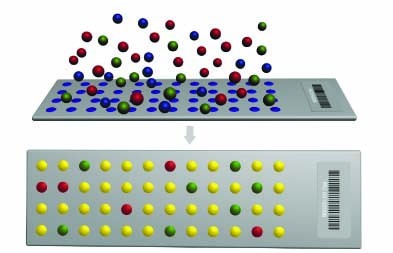The image depicts two oblong, silver, rectangular metal boards with numerous holes arranged in straight rows. The top board, which features blue and green spheres elevated in its airspace, is positioned horizontally halfway up the image, with some spheres appearing to bounce off its surface. A faint gray arrow in the center of the image points downward toward the second board. This second board is oriented vertically, facing the viewer, and contains various colored spheres—including yellow-green, green, and red—wedged into its perforations. Both boards, representative of comparative genomic hybridization arrays used in pathology, have a barcode visible on the right side. The scene highlights the transformation of sphere colors from green and blue on the top board to yellow-green and green as they settle into the board's grid, exemplifying genetic chromosomal analysis.